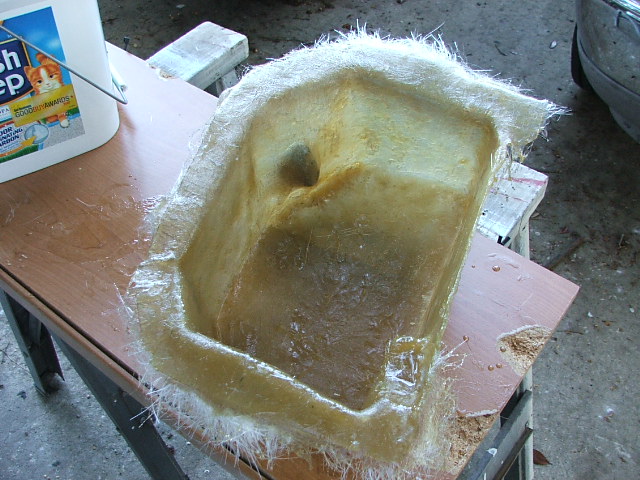The photograph depicts an indoor scene, likely set in a garage. The floor is made of gray cement and there's a makeshift table made from a brown laminate wood board supported by metal posts. The board is chipped, revealing the particleboard underneath. In the upper left corner of the image, there's a partially visible white plastic bucket identified as a Fresh Step Kitty Litter container with a label and an orange cap.

Dominating the right side of the scene is a fiberglass container, light honey-amber in color and rectangular in shape. This container looks old and worn, covered in white fuzz or cat fur, with frayed edges that make it unappealing to touch. It appears dirty and stained, giving it a rancid or moldy appearance, suggesting it has been in use for cat litter at some point.

In the upper right corner of the photograph, the front bumper of a silver vehicle can be seen, reinforcing the setting in a garage. The overall impression is one of neglect, with old, damaged items scattered around, possibly indicating an area used for storage or infrequently visited.